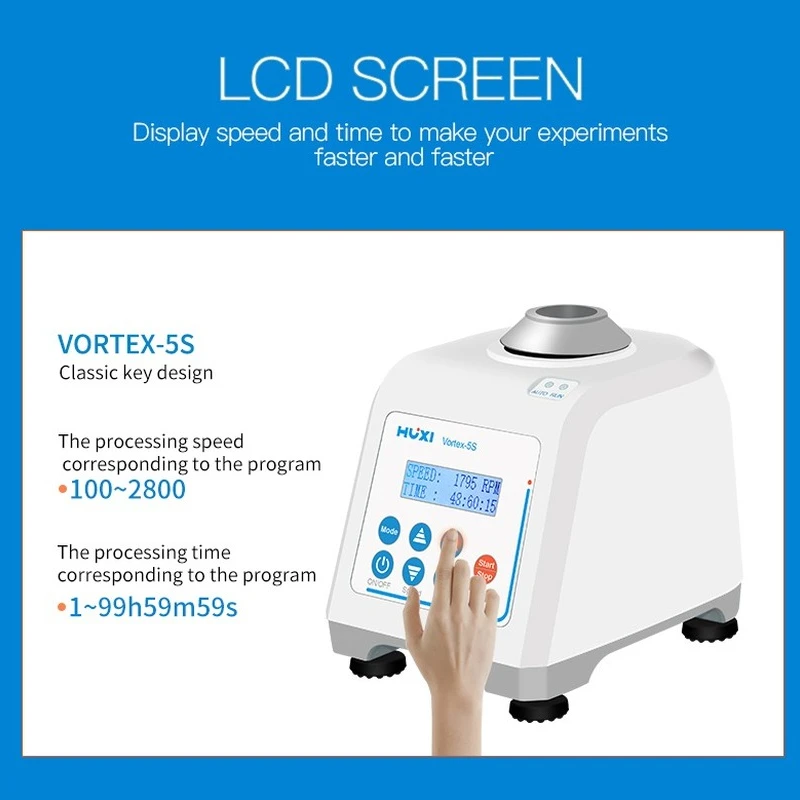The image is a highly detailed promotional print piece, with a predominantly blue border that is thick at the top and thin on the sides and bottom. The central background is white, formatted as a square. Blue and black text runs along the left side, containing key information. An LCD screen at the top displays the header "LCD screen" in large white font, followed by smaller text indicating functionalities: "Display speed and time to make your experience faster and faster."

In the main white rectangle, a square-shaped white device, labeled "HUXI VORTEX-5S" on its front, is prominently featured. The device stands on four black pedestal legs and has a silver-colored cylindrical component on top. There is a digital display screen with accompanying buttons on the front panel, and additional specifications note "VORTEX-5S classic key design," "Processing speed corresponding to the program 100-2800," and "Processing time corresponding to the program 1-99 hours 59 minutes 59 seconds." A Caucasian hand is seen engaging with the buttons on the device.